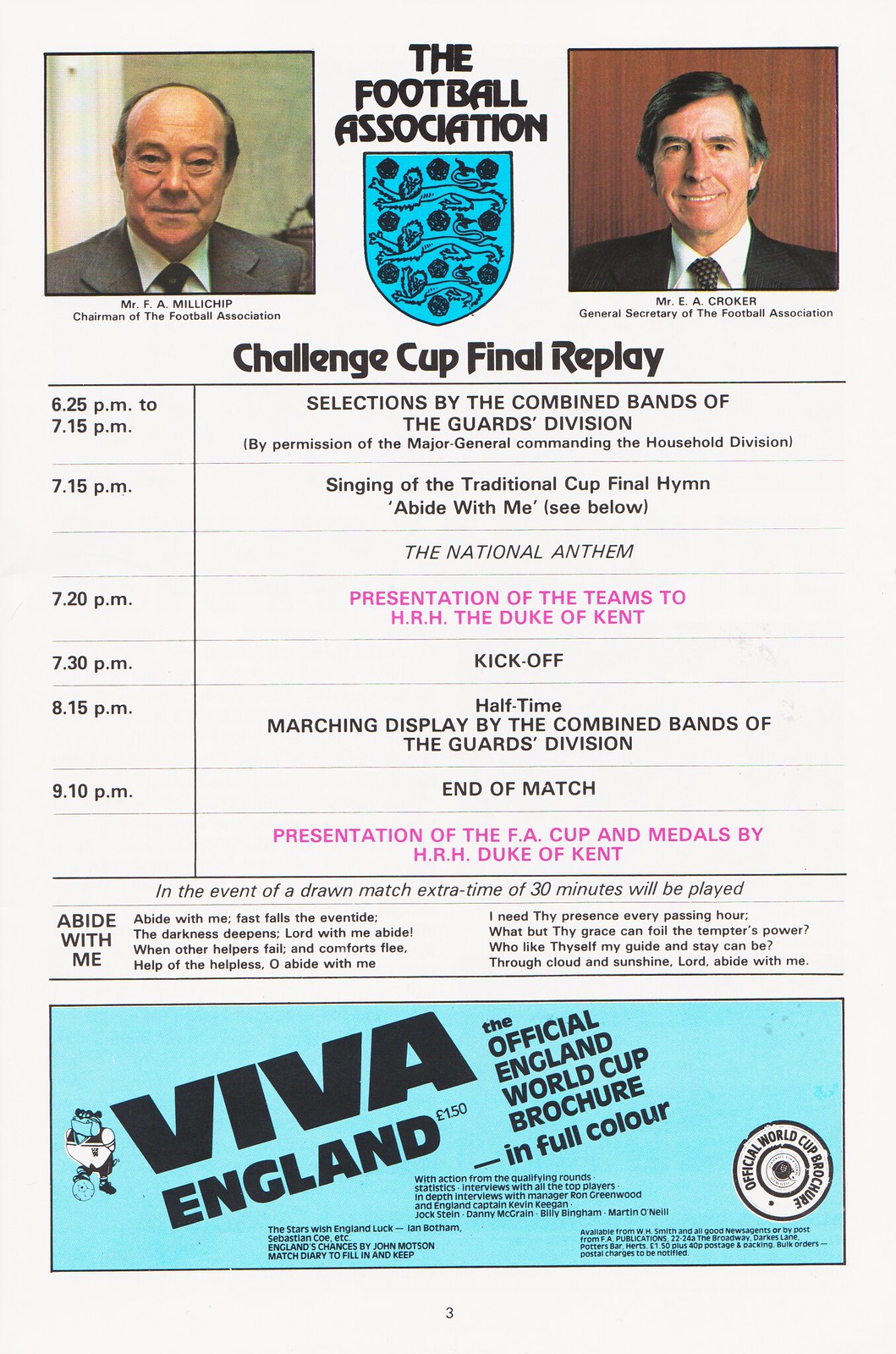The image depicts a rectangular paper with a gray background, prominently featuring content related to the Football Association Challenge Cup Final Replay. Centrally placed between two photographs is the heading "The Football Association" accompanied by a teal badge displaying sketches of monkeys chasing white round objects. 

On the left side of the paper, there is a picture of a man with a receding hairline, closed eyes, squinty brown eyes, dressed in a gray suit, white shirt, and black tie. The caption beneath identifies him as Mr. F.A. Melchep, Chairman of the Football Association. On the right side is another photograph of a man with predominantly black hair with touches of gray, smiling with visible teeth. His hair is parted to the right. This man's caption reads Mr. E.A. Croker, General Secretary of the Football Association.

Below the central heading, it says "Challenge Cup Final Replay" in bold font. Following this is a detailed schedule of the event, structured in a chart format with two columns. The left column lists times, starting from 6:25 PM and ending at 9:15 PM. The right column describes events: "Selections by the Combined Bands of the Guardians Division," "Singing of the Traditional Cup Hymn," "Presentation of the Teams," "Kickoff," "Halftime," "End of the Match," and "Presentation of the FA Cup and Medals by H.R.H. Duke of Kent," with certain items highlighted in pink.

The notice also includes a provision for extra time in the event of a draw, stating: "The Invent of a Draw Match, Extra Time of 30 Minutes Will Be Played." Below this, there are two columns of text with song lyrics titled "Abide With Me."

At the very bottom of the paper, there is a teal rectangle. On the left side of this rectangle, angled upwards to the right in black text, it says "Viva England, the Official England World Cup Brochure in Full Color." On the right side, there's a circle with a white background and black text that reads "Official World Cup Brochure." Additionally, there are three paragraphs of black text at the bottom of the paper providing further details.